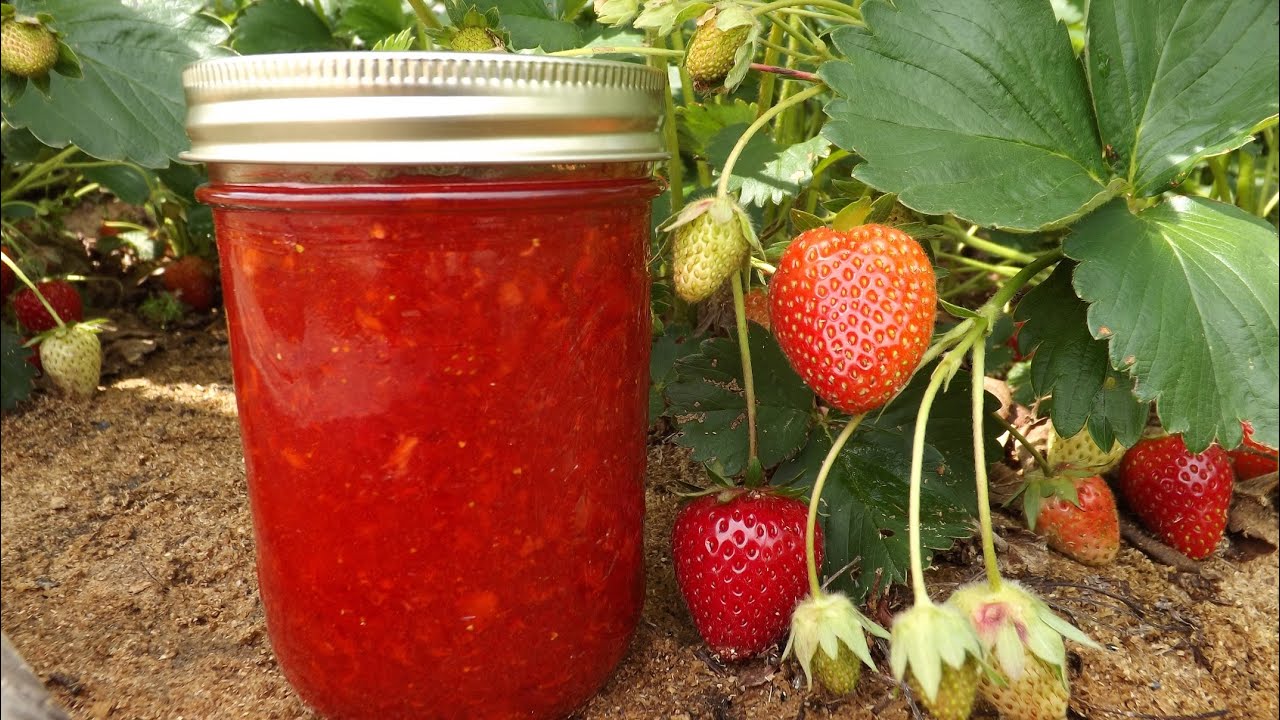This image captures a glass mason jar filled with bright red strawberry jam, complete with a metallic lid, placed on rich, fertile soil. Surrounding the jar are strawberry plants bearing fruit in various stages of ripeness, from lime green immature berries to partially ripened fruit and fully ripe, rich red strawberries. The strawberry leaves are lush and green, juxtaposing the vibrant red of the fruit and jam. The ground is earthy and sunlit, creating a cool and natural environment that highlights the total life cycle of strawberries, from initial growth to the final preserved product.